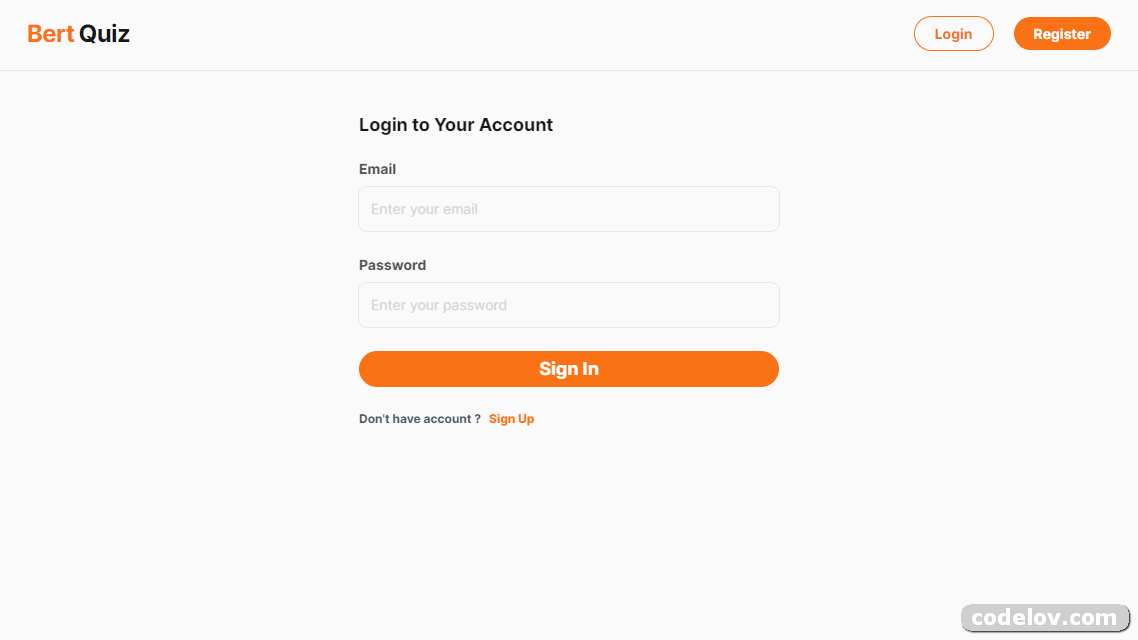An image displays a user interface for the BERT Quiz platform. In the top left corner, "BERT" is prominently written in orange letters, with "B-E-R-T" spelled out underneath. Below this, the word "quiz" is styled in black letters, "Q-U-I-Z". On the right side of the interface, there is a login button with orange text and a register button featuring white text on an orange background.

The central section prompts the user to log into their account. It includes fields for "Email" with an accompanying input box labeled "Enter your email" and "Password" with a box labeled "Enter your password". Below these fields is an orange button with the text "Sign In" in white letters, "S-I-G-N I-N". 

A message beneath the sign-in button reads, "Don't have an account?" in black text followed by "Sign up" in orange text. In the bottom right corner, the website's name "Codelov.com" is written, with "C-O-D-E-L-O-V" spelled out beneath.

The background of the interface is a white and gray gradient, and all other text elements are in black, maintaining a clean and minimalistic design.